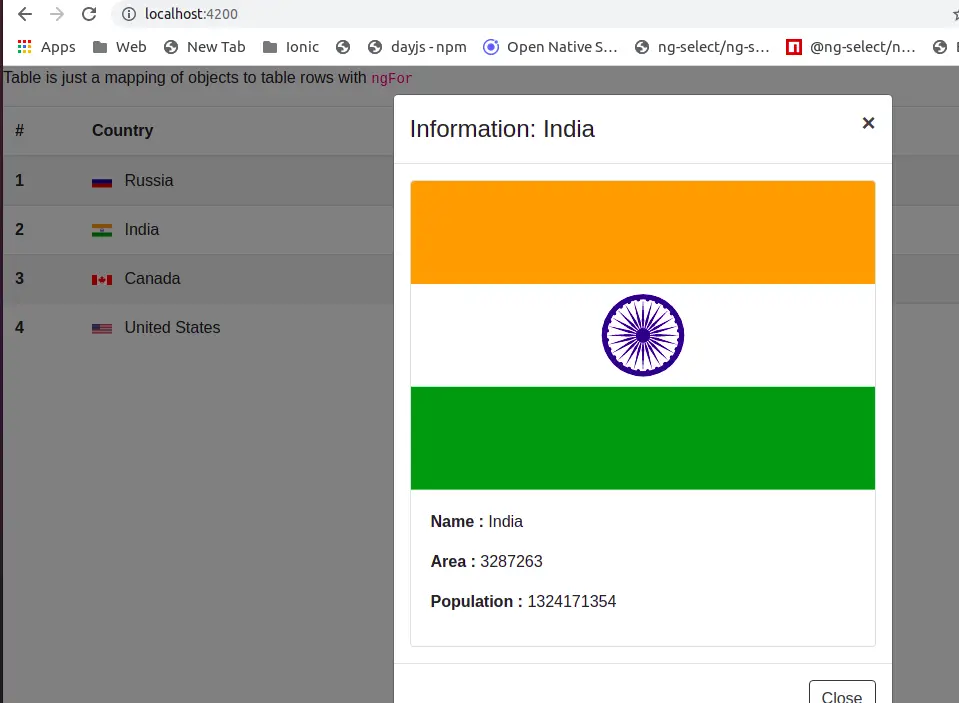Cropped screenshot of a website displaying statistical data about countries. The right and part of the left side of the webpage are cut off with a thin black line visible on the left side. The bottom portion is also cropped, missing any horizontal line or the full bottom view of the webpage. The browser address bar reads "localhost 4200."

In the main visible area, a large rectangular pop-up titled "Information: India" dominates the right side. Below the title, there's a prominent image of the Indian flag. Further down, the pop-up lists various details with notable labels: "Name: India," "Area: [Value]," and "Population: [Value]." At the bottom right of the pop-up, a white "Close" button with gray text is present, accompanied by a top-right corner "X" to close the box.

In the background on the left, partially visible, the webpage seems to display a table with headers "number" and "country" in bold black font. The list beneath includes four countries: "Russia," "India," "Canada," and "United States," with the United States listed fourth.